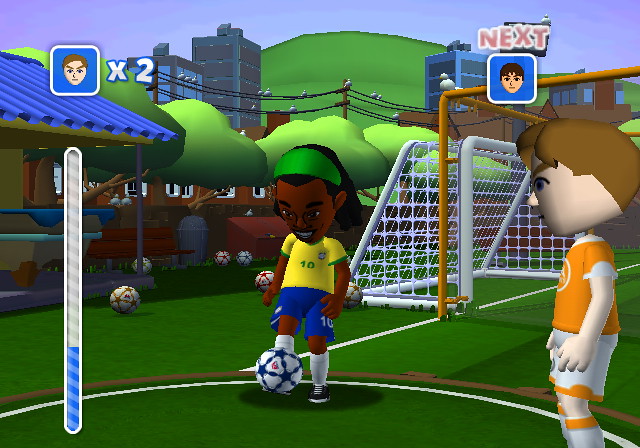This screenshot captures an intense moment in a soccer-themed video game set in an outdoor urban environment. The left-hand side of the image highlights a vibrant, bustling cityscape with tall buildings all around, power lines overhead, and seagulls perched elegantly on these lines. The playing field, enclosed by lush green trees at the outer edges, is adorned with a total of seven soccer balls – four red and three blue. A prominent blue bar at the bottom of the screen serves as a power meter, while on the right side, a player's avatar is displayed with a "x2" multiplier.

On the field, two players are engaged in play: one, a dark-skinned player with black hair decorated by a green band, wears a striking yellow jersey with the number 10, teamed with blue shorts, white socks, and black shoes. He is captured mid-action, kicking a blue and white soccer ball. Nearby, an opponent with brown hair, dressed in an orange jersey and white shorts trimmed with orange, complements his outfit with white socks capped by an orange band.

In the background, a classic white soccer goal with a white net stands guard, while the pitch itself is a vibrant green with crisp white markings defining the boundaries and key areas.